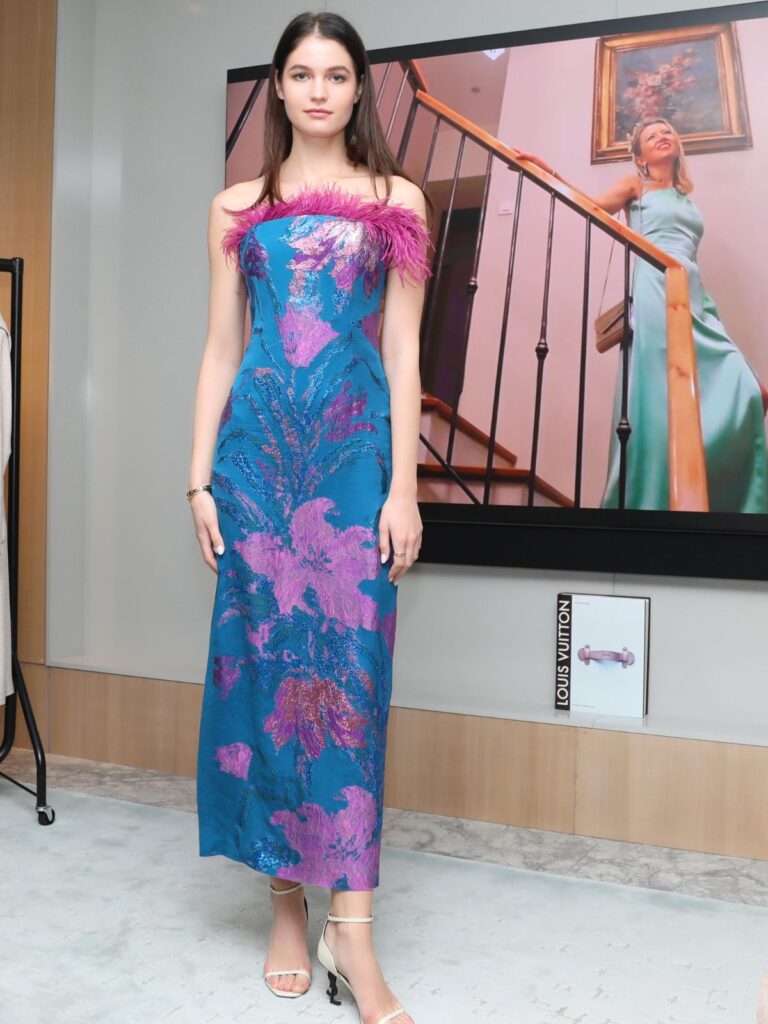The image depicts a young model in her early 20s posing for a full body shot. She has long, dark brown hair that flows over her shoulders, partially pulled back, and she wears a delicate bracelet on one wrist. Her dress, which accentuates her slender figure, is made from a linen-like fabric and features an abstract floral pattern with pink and purple flowers on a bluish-green base. A plume of pink, feathery material adorns the chest area of the dress, which is sleeveless and backless. On her feet, she wears warped white high heels. 

Behind her hangs a large photograph of a blonde woman descending a staircase. The woman in the photograph has shoulder-length hair and wears a long, silky blue dress, accessorized with red lipstick and a small brown purse on her right shoulder. A painting of flowers with a large frame appears just behind her head. Below this photograph, a shelf holds what appears to be a Louis Vuitton catalog. The model stands confidently, juxtaposing her own stylish presence with the fashionable scene depicted behind her.